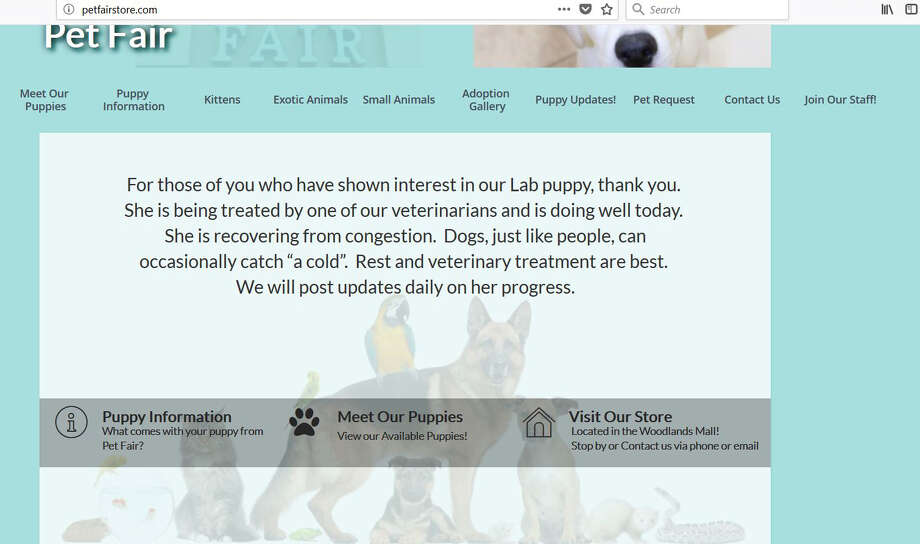The image appears to be a screenshot from a website dedicated to pets, identified by the text "Pet Fair" prominently displayed in the upper left corner. The background features a soothing blue-green gradient. To the upper right, there is a partial image of a dog, showcasing its nose, a portion of its white snout, and some tan fur. 

Beneath this, a navigational menu offers multiple clickable options, including "Meet Our Puppies," "Puppy Information," "Kittens," "Exotic Animals," "Small Animals," "Adoption Gallery," "Puppy Updates," "Pet Requests," "Contact Us," and "Join Our Staff."

Central to the image is a white-to-gray text box containing an update. The text reads: "For those of you who have shown interest in our lab puppy, thank you. She is being treated by one of our veterinarians and is doing well today. She is recovering from congestion. Dogs, just like people, can occasionally catch a cold. Rest and veterinary treatment are best. We will post updates daily on her progress."

In the background, you can faintly discern an image of a German Shepherd shot facing right but looking at the camera, with a parrot perched on its back. Lower in the image, there seem to be other animals, possibly including a puppy and a cat, though they are not distinctly clear.

A horizontal gray bar stretches across the picture of the animals, displaying text that reads: "Puppy Information," "Meet Our Puppies," and "Visit Our Store."